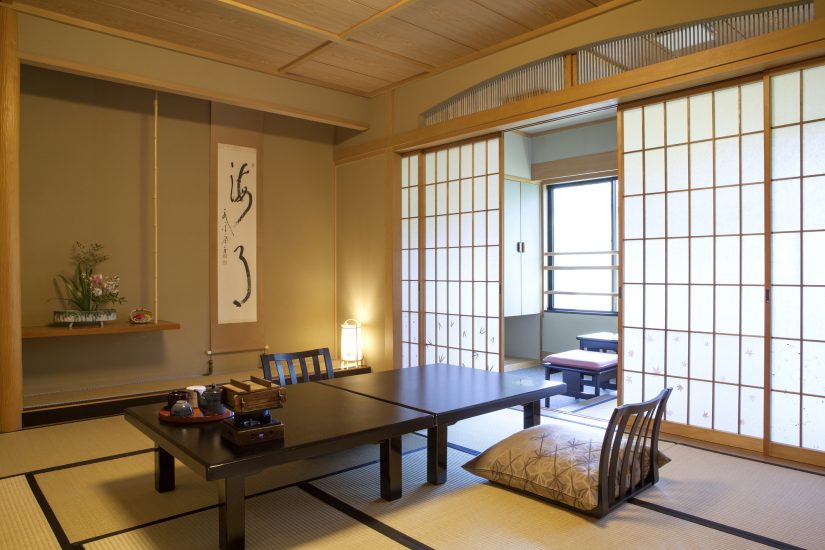This photograph captures the serene interior of a Japanese-inspired tea house. The room features very light-colored walls, separated by rice paper screen sliding doors. The central focus is a low, dark brown, cherry wood table, supported by eight legs. Accompanying the table are two floor-level chairs with taupe pillows and wooden backings designed for comfortable seating. A meticulously arranged tea set, consisting of a gray teapot and small cup, adorns one side of the table, while the opposite side remains free. The floor is covered with a rice paper-like material showcasing a subtle taupe and brown-striped design, enhancing the room's tranquil ambiance.

On the wall behind the table, a long and narrow piece of Japanese-inspired artwork is displayed, adding to the room's authentic character. To the left, a simple shelf hosts a delicate floral arrangement. The room extends into another space through the rice paper screen doors, revealing more low tables, cabinets, and windows that bathe the area in natural daylight. The secondary space features mustard-colored walls and a continuation of the minimalist aesthetic, further emphasized by an open window that connects the inside with the outside world. Warm light spills onto the floor, enhancing the inviting atmosphere of this meticulously arranged and elegantly simple space.